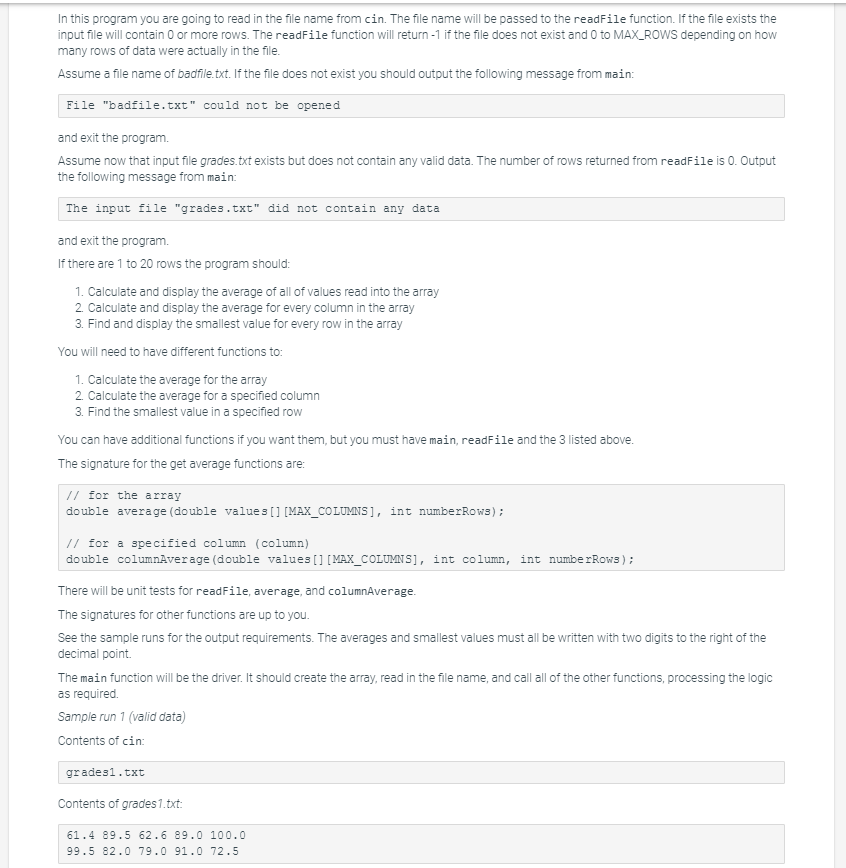This is a screenshot taken from an educational coding website focused on C++ programming. The image shows detailed information about a program designed to read filenames from user input via the console (stdin). The filename, once received, is passed to a function called `readFile`.

At the top, the documentation specifies that the program will read the filename from standard input (cin). If the specified file exists, the input file may contain zero or more rows of data. The `readFile` function will return -1 if the file does not exist or a value between 0 and `maxRows`, representing the actual number of rows in the file.

An example provided illustrates the case where the filename is "badfile.txt". If "badfile.txt" does not exist, the output should be: 

```
File "badfile.txt" cannot be opened
```

The program will then exit. 

Another scenario assumes an existing file named "grades.txt" which, although it exists, does not contain any valid data. If `readFile` returns 0 rows for "grades.txt", the program should output:

```
The file "grades.txt" did not contain any data
```

The program will then exit.

Additionally, the screenshot includes information on various other functions necessary for the program. These include functions to calculate the average of an array, column, or row, and to find the smallest value within the dataset. The image provides snippets of code and examples of expected outputs to guide the learner through implementing these functionalities.